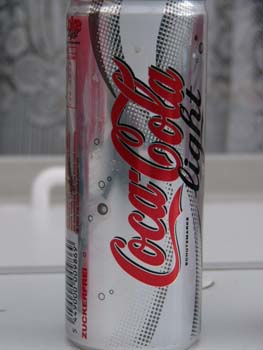The image features a tall, slender can of Coca-Cola Light prominently displayed on a white windowsill. The can is distinguished by its silver color and the classic Coca-Cola logo written in red, with the word "Light" positioned directly underneath in black, reminiscent of Diet Coke branding. The can is adorned with a subtle design consisting of black, gray, and darker gray dots that extend across its surface. In addition, a barcode and ingredient list are visible on the side of the can. Behind the can, net curtains drape over the window, complementing the overall scene, with hints of gray patterned wallpaper in the background, contributing to the image's domestic and relaxed atmosphere.